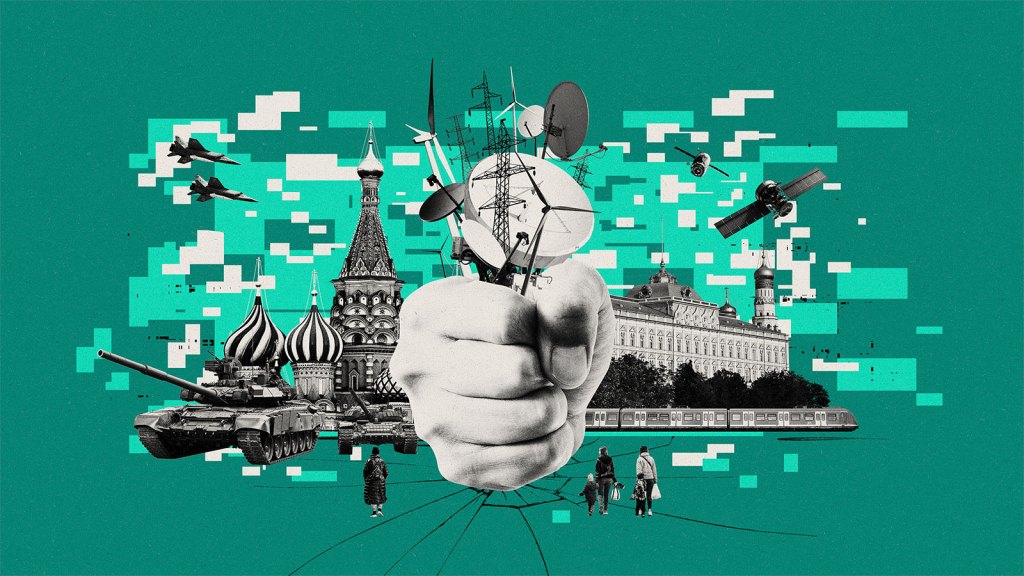This stylized digital artwork features a greenish-teal background with pixelated patterns in lighter green and white. The central focus is a large black-and-white fist slamming into the ground, creating cracks that spread outward. The fist is gripping various communication devices, including antennas, satellites, radio towers, and a wind turbine. Surrounding this powerful image are grayscale depictions of military and Russian imagery: a tank in the bottom left, fighter jets in the top left, and notable architectural structures like the Kremlin and a chapel-like building, with a large square-shaped building on the right. Smaller, indistinct civilians walk from the bottom of the image toward the center, dwarfed by the towering fist and buildings. The overall digital composition suggests themes of power, conflict, and possibly protest, highlighted by the contrast between the greenish-teal background and the stark black-and-white imagery.